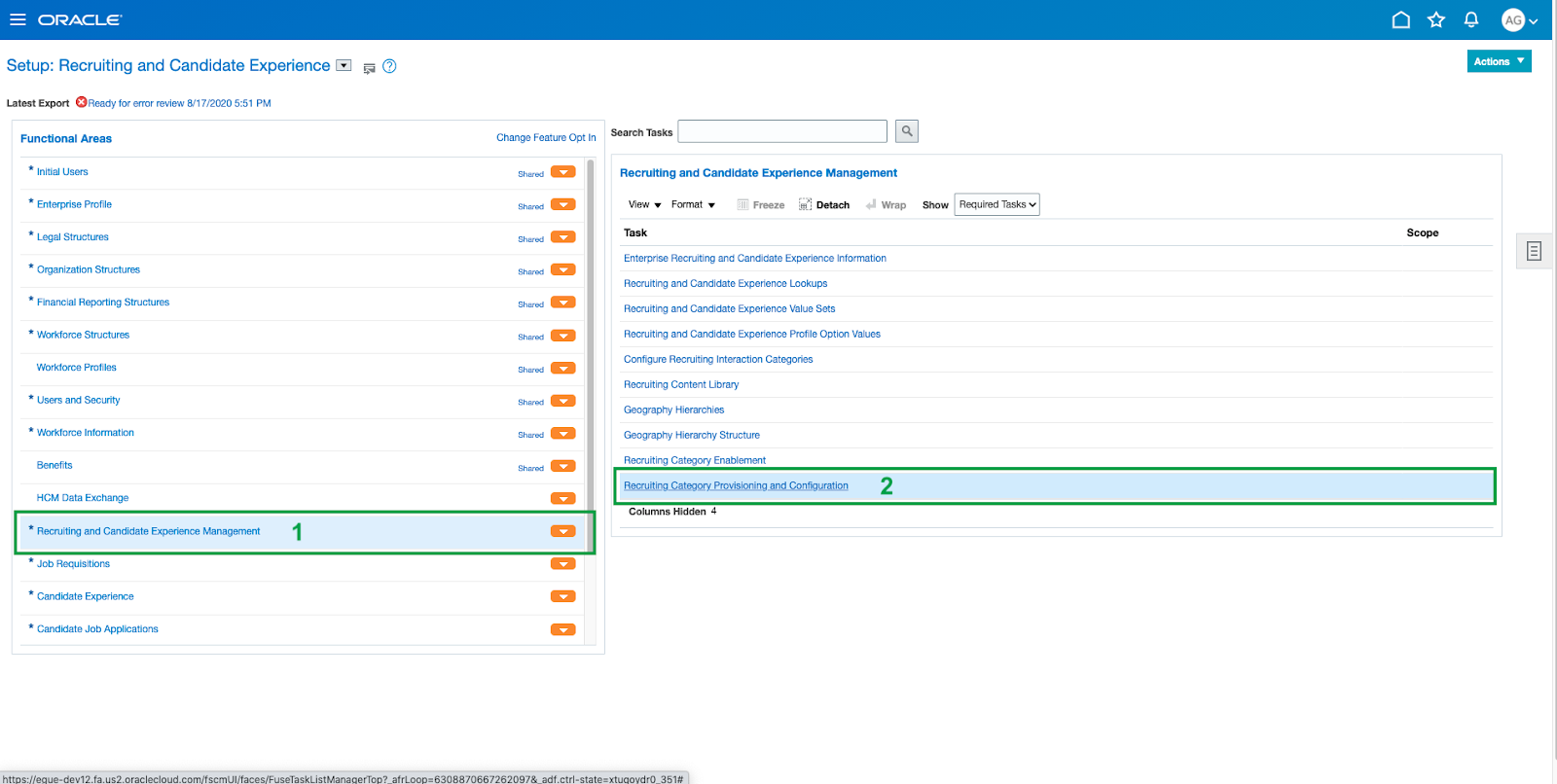This is a detailed screenshot of a tab within Oracle's Performance Management software. At the top, a blue bar houses the Oracle logo on the left, and a menu bar adjacent to it. On the right side of the blue bar, there are icons for home, favorites, alerts, and user profile, followed by a drop-down menu next to the profile icon. The main body of the page, set against a white background, begins with the labels "Setup," "Recruiting," and "Candidate Experience" on the top left.

A substantial tab on the left side is titled "Functional Areas," featuring a vertical list of items. Each item on the left is paired with an orange "Setup" button on the right. Midway down this list, there is a green-edited box highlighting the "Recruiting and Candidate Experience Management" section, marked as step one on the image. On the right panel, another highlighted section includes "Recruiting Category," "Provisioning," and "Configuration," marked as step two. The green rectangles and numerical annotations are guides indicating the order of operations: first, click on the relevant left-side item, which opens the setup options in the right panel, then proceed to select the necessary options in the "Recruiting Category," "Provisioning," and "Configuration" section.